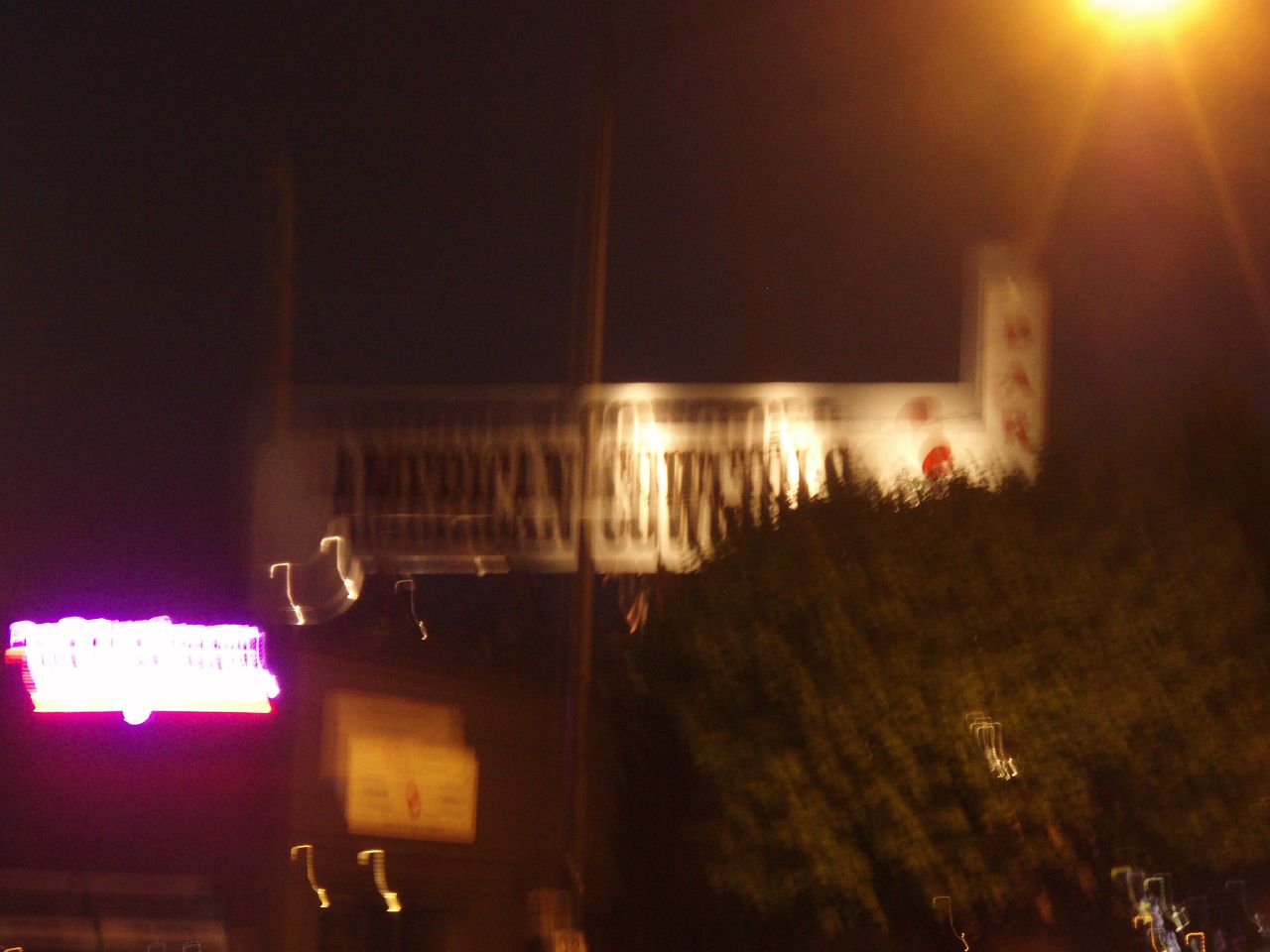A slightly blurry, out-of-focus nighttime photograph captures the vibrant façade of a building marquee. In the lower left-hand corner, a pink neon sign glows brightly, casting a warm hue against the dark backdrop. The upper right-hand corner of the image features the intense yellow-white glare of a streetlight, contrasting sharply with the darkness. A fluffy green tree occupies the lower right-hand quadrant, its leaves faintly illuminated by the ambient light. Central to the photograph is a partially lit white marquee, displaying the partially discernible text, "American Cow...," with the word "BAR" written vertically at the end.